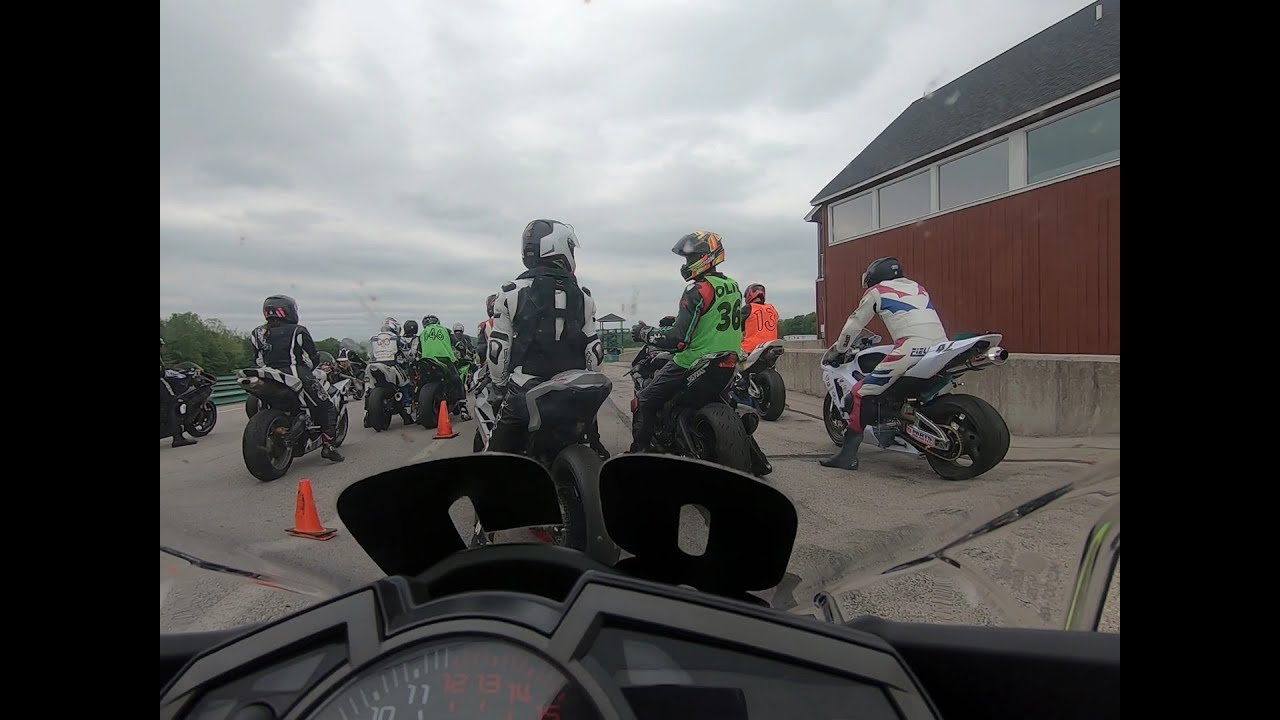The image depicts a scene from the perspective of someone seated on a motorcycle, likely taken from the dashboard which includes a speedometer and a mirrored number, appearing to be either 58 or 68. Vertically aligned black bars frame either side of the image. In front of the camera, a group of motorcyclists is preparing for what appears to be a race, evident from the lining up and presence of orange traffic cones on the ground. The riders sport a variety of vests and helmets, with one individual in a green vest marked with the number 36 and another in an orange vest with the number 13. The helmets, mostly dark, create a cohesive visual despite the different vest colors. To the far right of the image, a red barn-like structure with a black roof stands out against a cloudy sky. The setting seems to be a cement raceway, adding a sense of anticipation and competitive spirit to the scene.